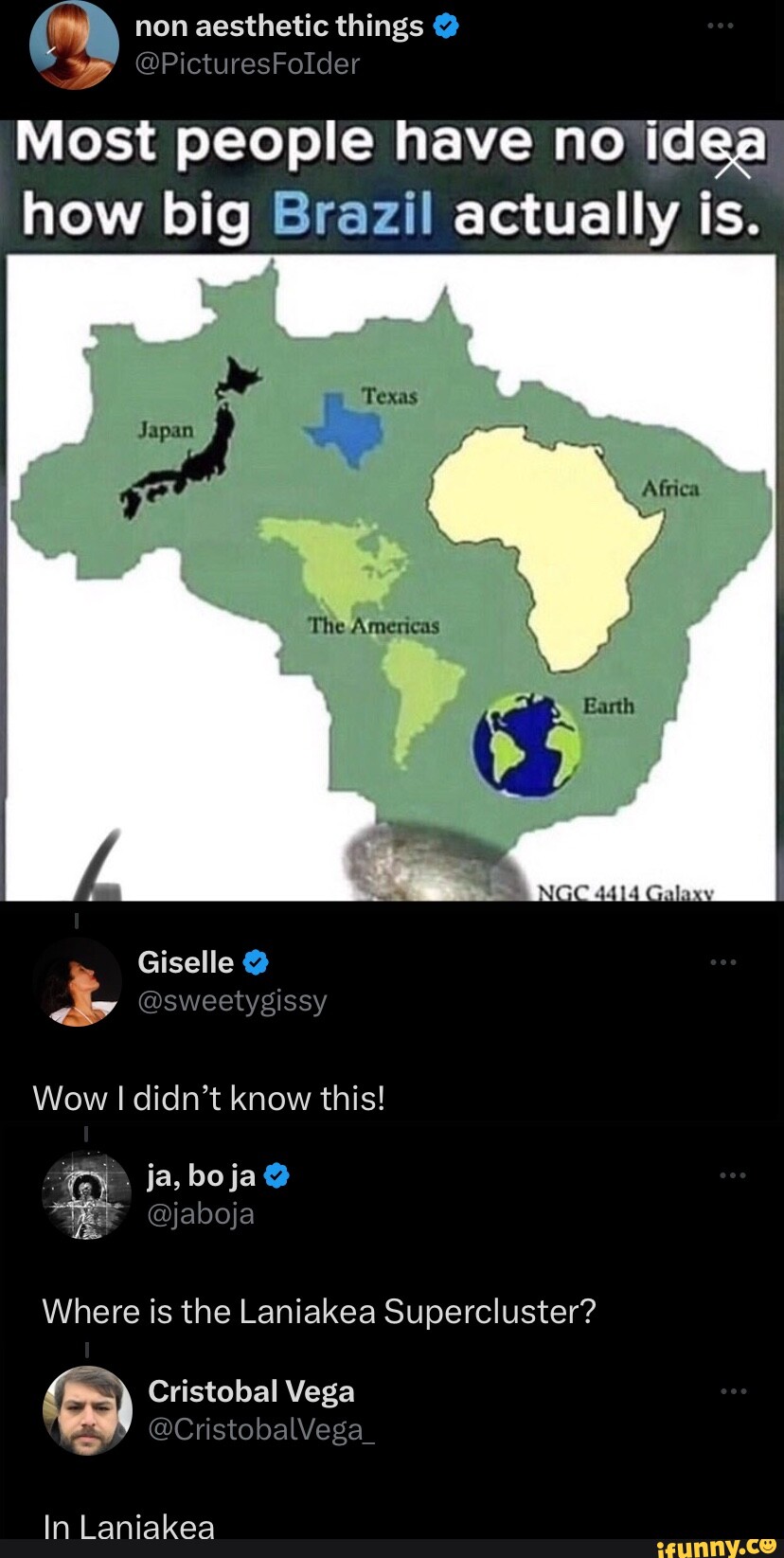Here is a cleaned-up and detailed caption for the provided image description:

---

**Image Description:**

The image is a composite meme featuring a screenshot from Twitter and is presented against a black background. 

**Top Left Corner:** 
- A profile picture of a woman with blonde hair partially covering her face.
- The username "non-aesthetic things" is displayed in white text.
- Below the username, a gray checkmark icon is visible.

**Below Profile Image:** 
- A grayish background with the text "Most people have no idea how big Brazil is," where the word "Brazil" is highlighted in a baby blue color.
- Underneath, there is a depiction of a map of Brazil, filled with various geographic entities: Japan, Texas, Africa, the whole of the Americas, and even the Earth itself.

**Right Side:** 
- A second profile picture of a supermodel, who is presumably Gisele Bündchen, looking up to the right.
- The username "Gisele" followed by a blue checkmark and the handle "@Sweetie" or "@SweetGissy" are displayed in a smaller gray font.
- White text below this reads, "Wow, I didn't know this."

**Bottom Left Dialogue:** 
- A user named "Jabaja" asks, "Where is the Sri Lankan Super Custard?"
- Another user, "Christabel Vega," responds, "In Sri Lanka."

**Bottom Right Corner:** 
- The iFunny watermark, "ifunny.co," is displayed in yellow text.

---

Overall, the image is a humorous take, blending a Twitter exchange with a map visual to emphasize the surprisingly large size of Brazil, complemented by an entertaining and somewhat nonsensical dialogue about Sri Lankan Super Custard.